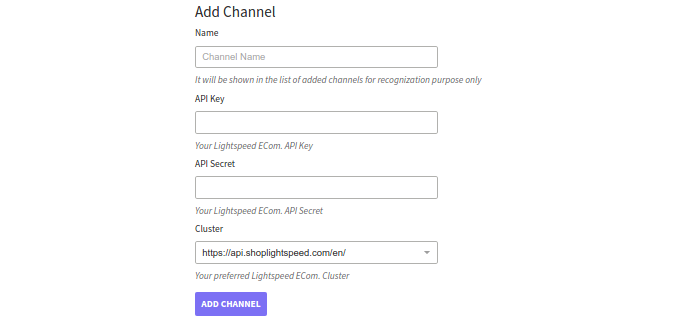The image depicts a minimalist interface for adding a new channel to a website or application. The design is straightforward, featuring a white background with black or dark gray text, ensuring readability and simplicity. 

At the top, there is a prominent header labeled "Add Channel." Below the header, the form comprises several elements designed for user input. The first input field is labeled "Name," with an accompanying text box pre-filled with the placeholder "Channel Name." This field is meant for users to identify the channel in their list of added channels; it specifies that the name is for recognition purposes only.

Next, there are two input fields related to API integration: "API Key" and "API Secret," both of which are empty text boxes. These fields are meant for users to input their Lightspeed Ecom API credentials, ensuring secure access to the service.

Further down, a dropdown menu titled "Cluster" allows users to select their preferred Lightspeed Ecom cluster. The dropdown is currently set to "https://api.shoplightspeed.com/en." 

At the bottom of the form is a striking purple button with white text that reads "Add Channel," providing a clear call-to-action. The interface’s overall design maintains consistency with minimal color variation, using white, black, and dark gray, while the only accent color is the purple of the action button, drawing attention to it.

The layout is uncluttered and functional, emphasizing input accuracy and simplicity for ease of use.